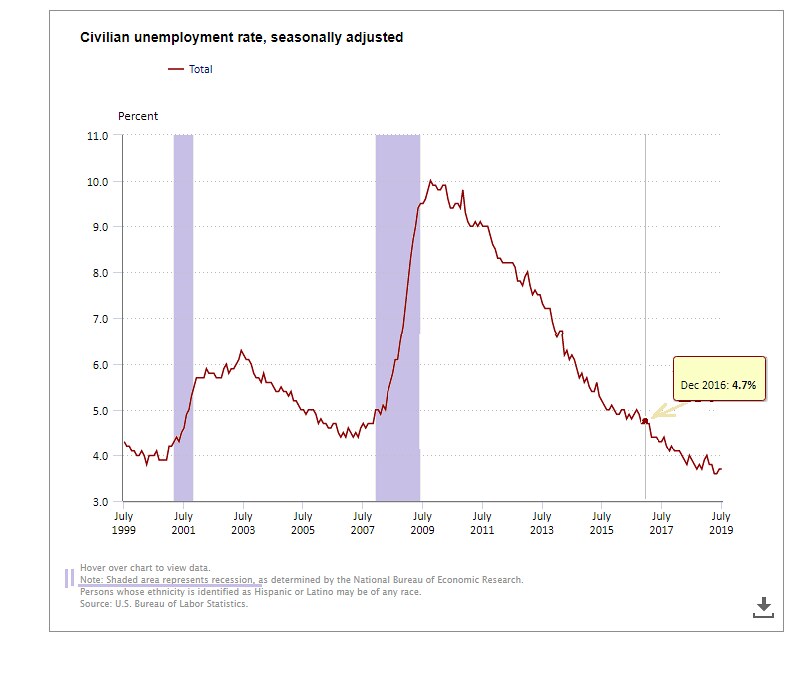The image displays a square white graph chart titled "Civilian Unemployment Rate, Seasonally Adjusted" in small letters at the top left. Below the title, a red line labeled "total" tracks unemployment trends over time. The vertical axis on the left is marked with percentages from 3.0% to 11.0%, and it is labeled "percent" in small black letters. The horizontal axis spans from July 1999 to July 2019, marking years at two-year intervals. The red graph line begins near 4.0% in July 1999, rises sharply to a peak of around 10.0% by July 2009, then gradually declines back to below 4.0% by July 2019. Notable features include two thin purple vertical bars: one above July 2001 and another between July 2007 and July 2009. According to an annotation at the bottom, "hover over the chart to view data," with additional text noting that no shaded area indicates recession periods as determined by the National Bureau of Economic Research.